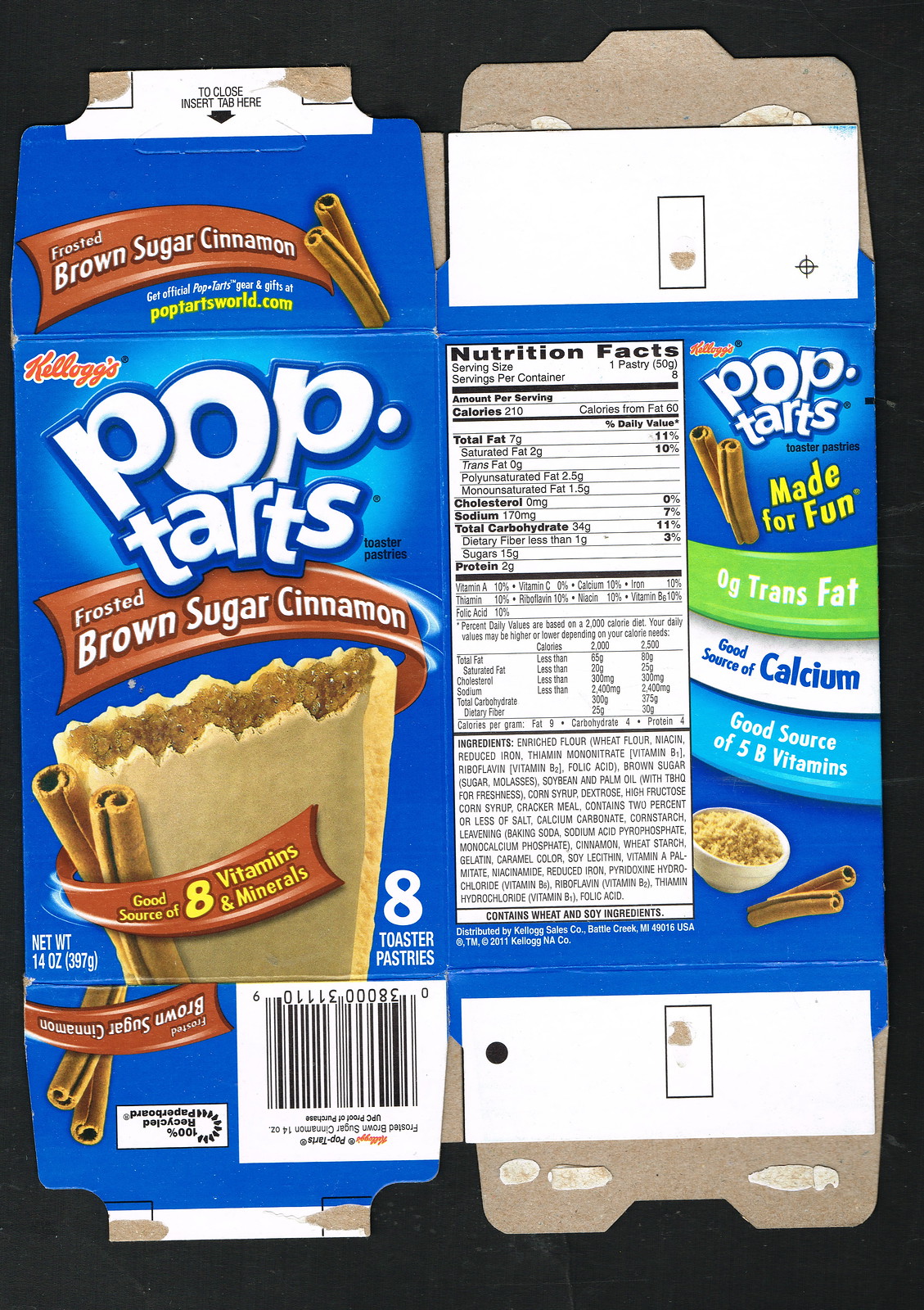The image features a flattened cardboard box of Kellogg's Frosted Brown Sugar Cinnamon Pop-Tarts. The design allows the front and back panels to be viewed simultaneously. 

The front cover, predominantly brown, displays the Kellogg's logo in the top left corner. The prominent Pop-Tarts logo sits across the top in white font. Below, the description "Frosted Brown Sugar Cinnamon" is visible, accompanied by an image of a bitten-into Pop-Tart with a light brown exterior and a darker brown interior. To the left of the Pop-Tart, two whole cinnamon sticks are prominently displayed, emphasizing the flavor. Additionally, this section mentions that the product is a good source of 8 vitamins and minerals.

On the back of the box, the Nutrition Facts panel is clearly labeled, detailing the nutritional information. To the right of this panel, the text "Pop-Tarts made for fun" is evident, highlighting key health information such as zero trans fat, a good source of calcium, and a good source of five B vitamins. A white bowl, possibly for cereal, with two cinnamon sticks lies next to this text. The box's bottom flap, which is scalloped rather than torn, features an upside-down barcode.